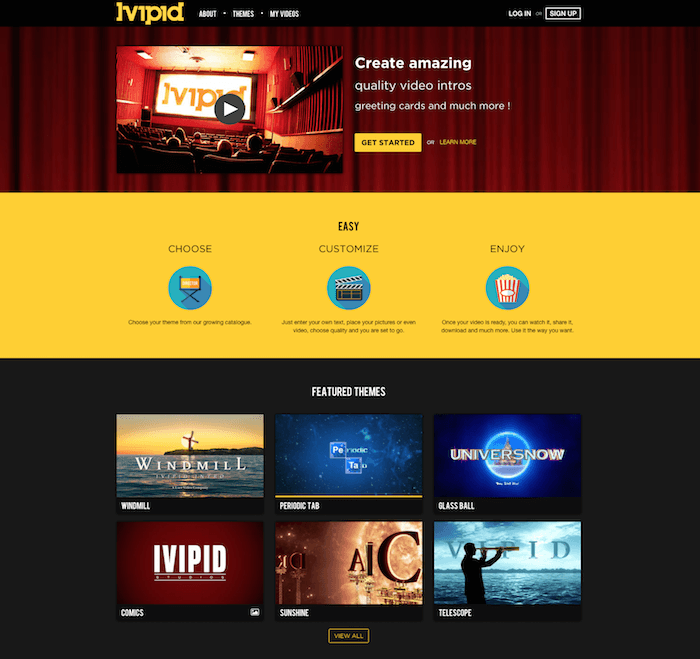This descriptive caption should provide a clear picture of the webpage:

---

This is a screenshot from the website Evipid. The brand name "Evipid" is prominently displayed in yellow block letters within a black header. To the right of the name are tabs labeled "About," "Themes," and "My Videos," all aligned in a row. In the top right corner, there are "Login" and "Sign Up" buttons. Below the header lies an image depicting a movie theater screen, framed by a cinema curtain, displaying the "Evipid" name. To the right of this image is a text block that reads, "Create amazing quality video intros, greeting cards, and much more," followed by a yellow "Get Started" button and a "Learn More" link. 

Beneath the picture, a white and yellow banner with the word "Easy" in the center is displayed. The banner features three icons: a director's chair labeled "Choose" on the left, a clapperboard labeled "Customize" in the middle, and a popcorn box labeled "Enjoy" on the right. The bottom section of the webpage has a black background and a title that reads "Featured Themes." Here, six screenshots are showcased. The first screenshot is titled "Windmill," depicting a windmill at the edge of a landmass surrounded by water. The last screenshot, located on the bottom right, is labeled "Telescope," showing a man looking through a telescope over the ocean. At the bottom center of this section, there is a "View All" button. 

---

This detailed caption provides a comprehensive visual representation of the Evipid webpage.